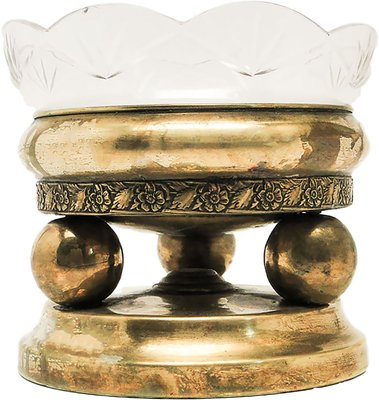This color photograph, in portrait format, showcases an intricate and mysterious metallic object, appearing ancient and somewhat rusted. Suspended in a white background, the object has a distinctive layered design. At the top, there is a white, puffy, cushion-like shape reminiscent of a couch, this element appears to be ornamental. Beneath it is a gold band encircling the object. Directly below this band is another gold band adorned with floral designs, featuring seven visible flowers wrapped around its circumference.

Supporting this section are three brass, marble-like spheres, which hold up the floral band. Below these spheres, another brass ring acts as a base for the entire structure. The object reflects light, hinting at the photographer's presence, and while it gives a sense of antiquity, its function remains unclear. The object’s top section is glass-like with humps along the edge, suggesting it might be some sort of decorative glass bowl. The combination of materials and elaborate design makes it a unique and perplexing piece.